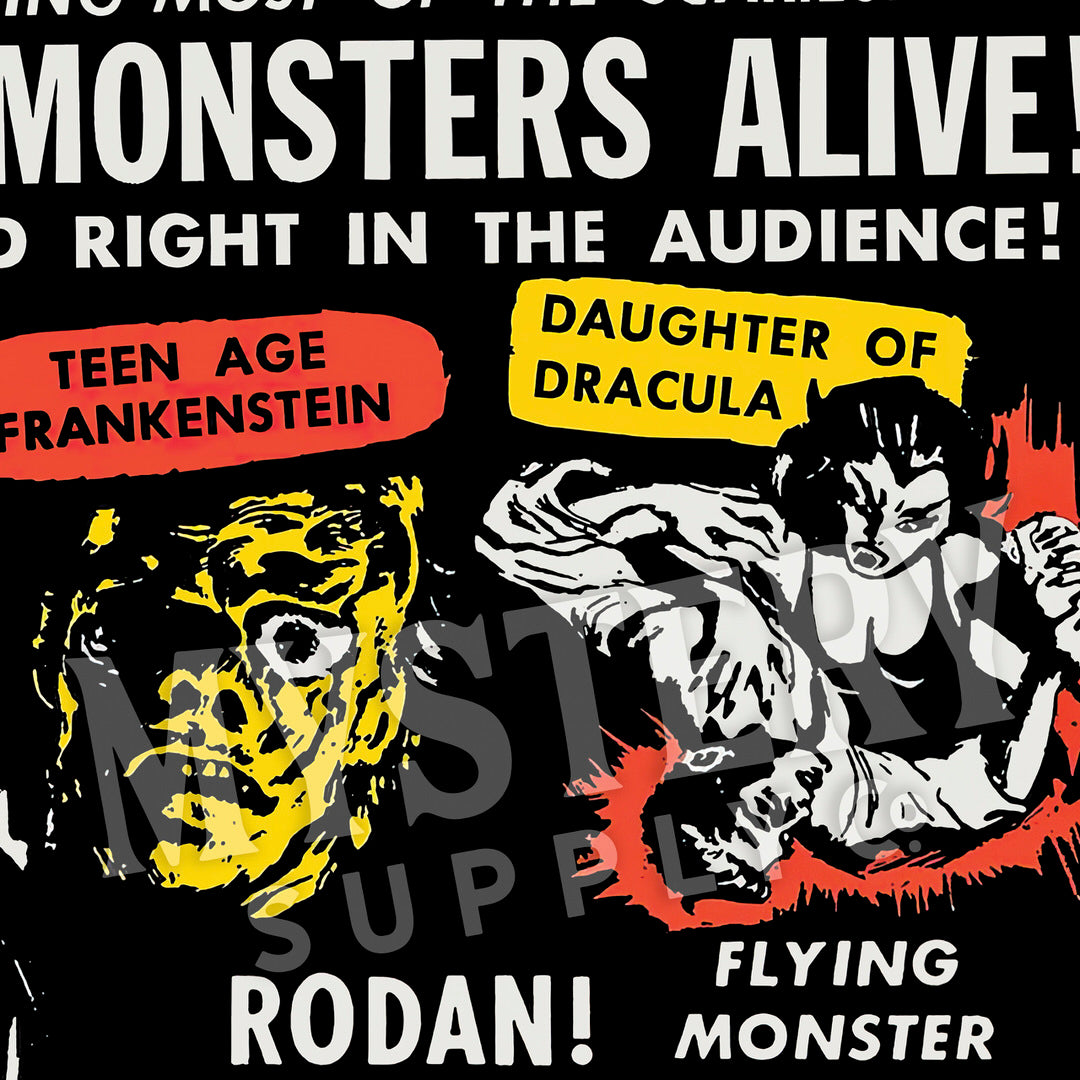The image is a cropped section of a vintage, cartoon-style movie poster. It prominently features bold text, "Monsters Alive! Right in the Audience!" accompanied by exclamation points. On the left side, there's an orange text bubble that says "Teenage Frankenstein" with a partial yellow image of Frankenstein's face, his features partly obscured in shadow. To the right, a yellow text bubble reads "Daughter of Dracula" and shows a pale-skinned woman with black hair, seemingly about to bite a man's neck. At the bottom of the poster, the text states "Rodan, Flying Monster!" further suggesting a kaiju appearance. The overall composition hints at an audience-engaging, fictional cinematic event or a themed t-shirt design, blending classic monster film elements.